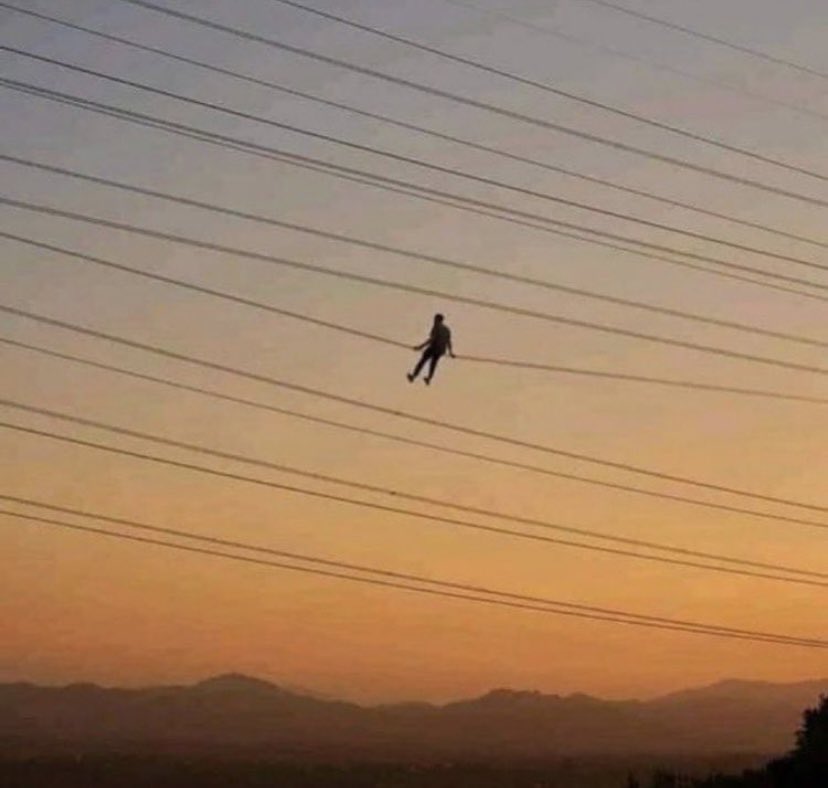In this surreal and slightly unsettling image, a man sits alone on thin, high wires that stretch diagonally upwards from the right to the left, creating a stark contrast against the vibrant twilight sky. The man is silhouetted, with his feet outstretched in front of him and his hands gripping the wire for balance, causing the wire to sag slightly under his weight. The sky behind him transitions from a light purple at the top to a deep orange near the horizon, further enhancing the dreamlike quality of the scene. Below the wires, a dark brown landscape with rolling, jagged hills adds depth to the composition, while a lone tree's silhouette in the bottom right corner anchors the image. The overall effect is one of isolation and intrigue, evoking a sense of wonder about the man's predicament high above the earth, surrounded by the fading light of day.